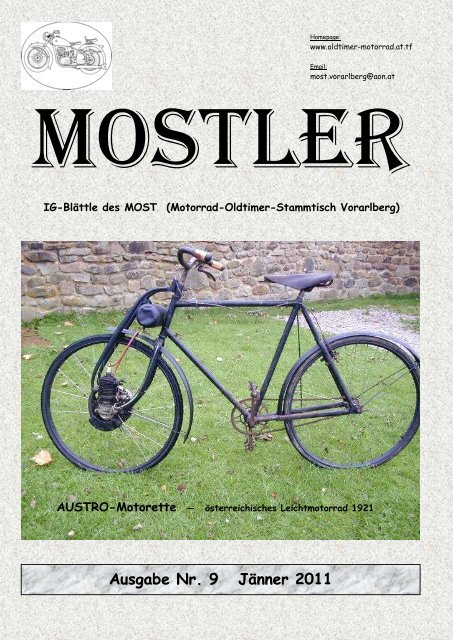The cover of the magazine, titled "Mosler" in a gothic black font with a white border, features a detailed and nostalgic theme. Against a gray backdrop and a brick wall in the background, an illustrated motorcycle occupies the upper left corner. Prominent beneath the title are several lines of text in a foreign language. Centrally located on the cover, a well-worn black 10-speed bicycle with a small motor mounted on the front tire stands upright on a lush green grass field. Additional foreign text is visible below the bicycle. Near the bottom, a rectangular section highlights "Oski in R9, January 2011." Colors on the cover include shades of gray, white, black, brown, and green, contributing to its vintage appearance.